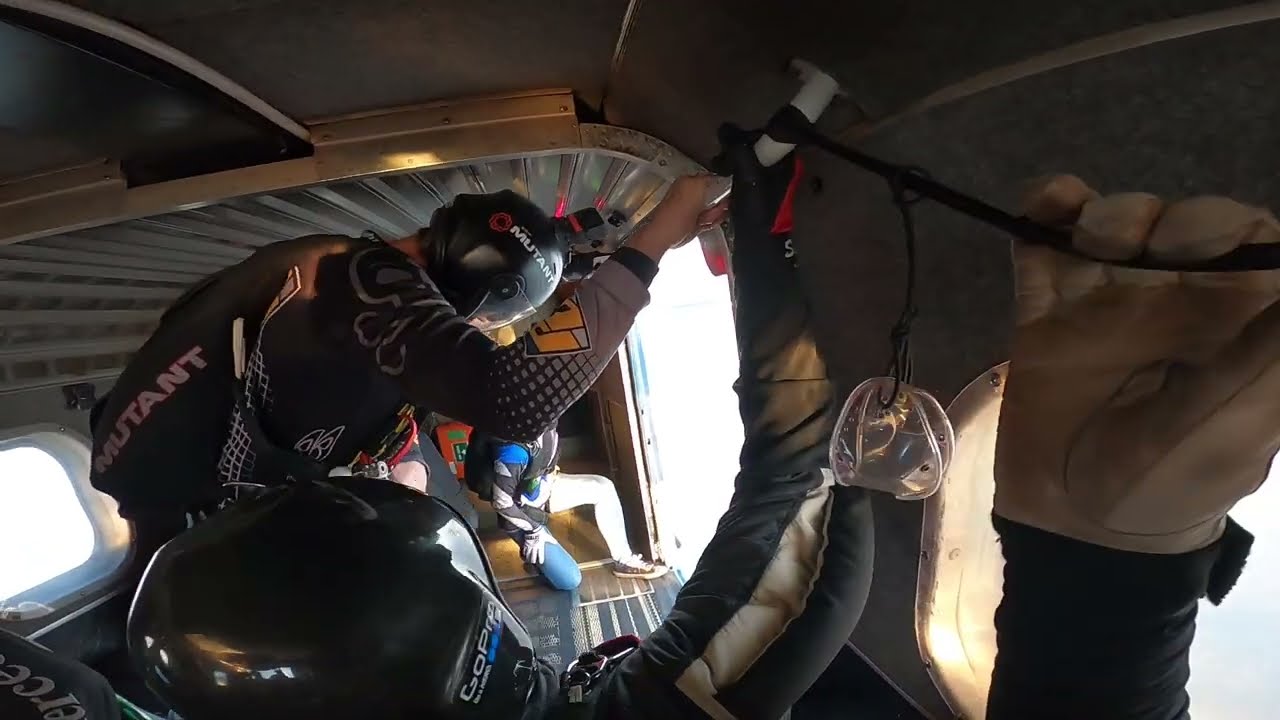Inside the airplane, a group of individuals is preparing to jump out, creating a scene charged with tension and anticipation. The plane's open door on the right side frames the vast sky outside, bathed in bright light that contrasts sharply with the dim interior. At the door stands a person in a black and gray long sleeve shirt, emblazoned with the word "MUTANT," which is also printed on their black parachute and black helmet. They peer down, visor down, seemingly ready for the leap. Nearby, another individual kneels on one knee in a black parachute, blue pants, and a blue, black, and gray jacket, poised to follow. In the foreground, a third person holds tightly onto a white handle on the ceiling, wearing a white and black jacket and a black helmet, clearly bracing for their turn. On the very left, the plane’s curved ceiling presses close to their heads, necessitating a stooped posture, while a glaring light enters through a small window at the bottom, hinting at the bright expanse outside. Amidst them, scattered black cords and ropes dangle, adding to the sense of organized chaos as they prepare for the exhilarating jump.